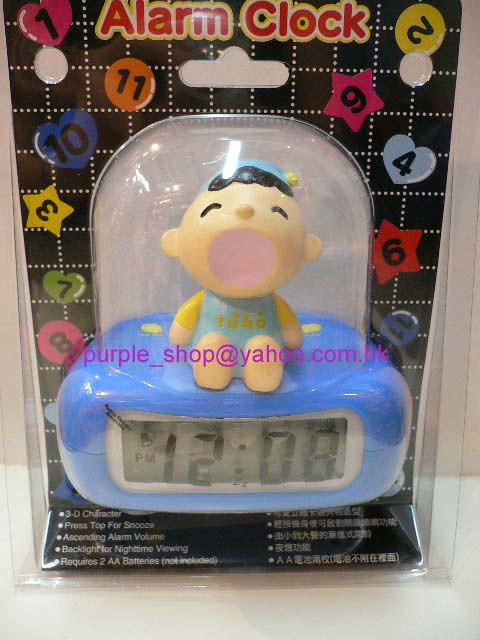A detailed photograph showcases a whimsical blue alarm clock still encased in its original plastic blister packaging. The clock, placed on a pristine white surface against a matching white background, features a playful, curvy blob shape. Atop the clock sits a charming cartoon character—an exuberant boy dressed in a blue shirt with contrasting yellow sleeves. His design is marked by a big round head, closed eyes, and exaggerated features, capturing a moment of mid-yawn with his mouth wide open and arms stretched upwards. His bare toes peek out, adding to the figure's endearing simplicity and cuteness. The black top of the packaging prominently displays the text "Alarm Clock," surrounded by a scattered array of numbers, emphasizing its function while maintaining the playful theme.